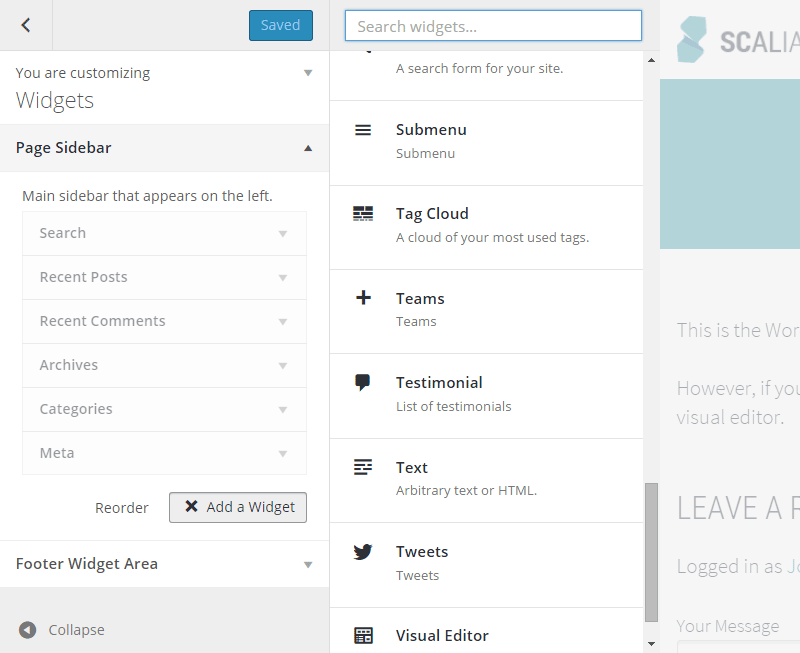The image depicts a composite of multiple webpage screenshots, organized into distinct panels, resembling a complex dashboard interface. On the left panel, there's a customization tool for widgets with options for adjusting the 'Page Sidebar' and 'Main Sidebar.' The title reads "You are customizing widgets," suggesting the user can add and personalize elements on a webpage. A reference is made to a 'Footer Widget Area' which seems to extend partially out of view.

The central panel showcases a search bar for finding different widgets. Even without input, a list of various widget options is visible, highlighted in alphabetical order. The list includes items such as 'Submenu,' 'Tag Cloud,' 'Teams,' 'Testimonial,' and continues through to 'Tweets' and 'Visual Editor,' indicating the breadth of customizable features available to the user.

On the right side of the image, a partial screenshot appears to contain text related to 'Scalia,' potentially referencing a relevant application or tool, though the details are partially obscured. This detailed layout suggests a robust interface for web design and customization, providing users with a myriad of options to enhance their webpage functionalities.